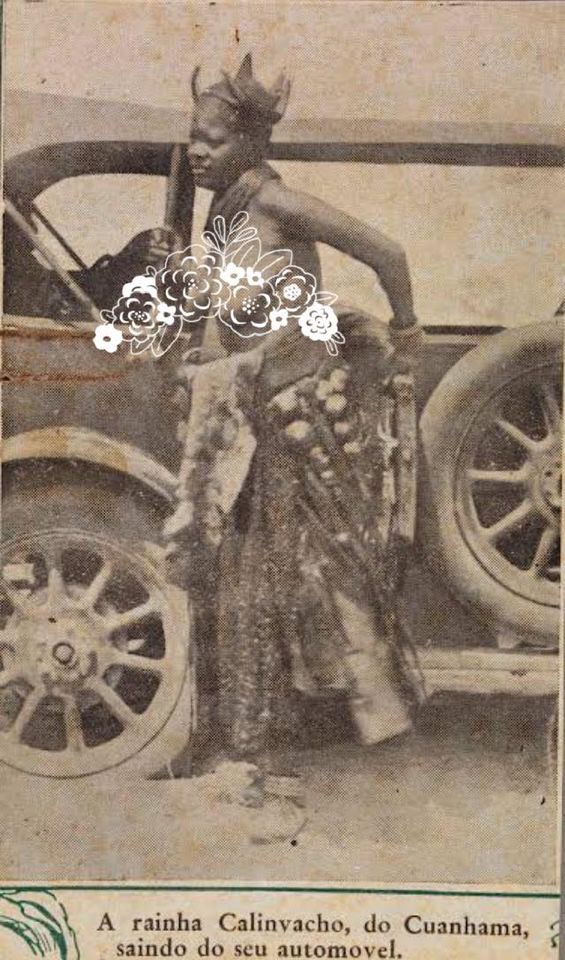This black-and-white newspaper clipping appears to be from the early 1920s and prominently features a topless African woman, though her upper body is partially obscured by a white floral pattern. She is clad in traditional dress on her lower half, which includes various tools and possibly fur, and is posed beside an old-school vehicle. The car, distinctive for its era with fabric top and a spare wheel attached to its side, lacks visible windows. The woman is standing by the passenger door, facing left, and there are no other individuals present in the image. Beneath this historic scene, the image is captioned with text in a foreign language, most likely Spanish or Latin.